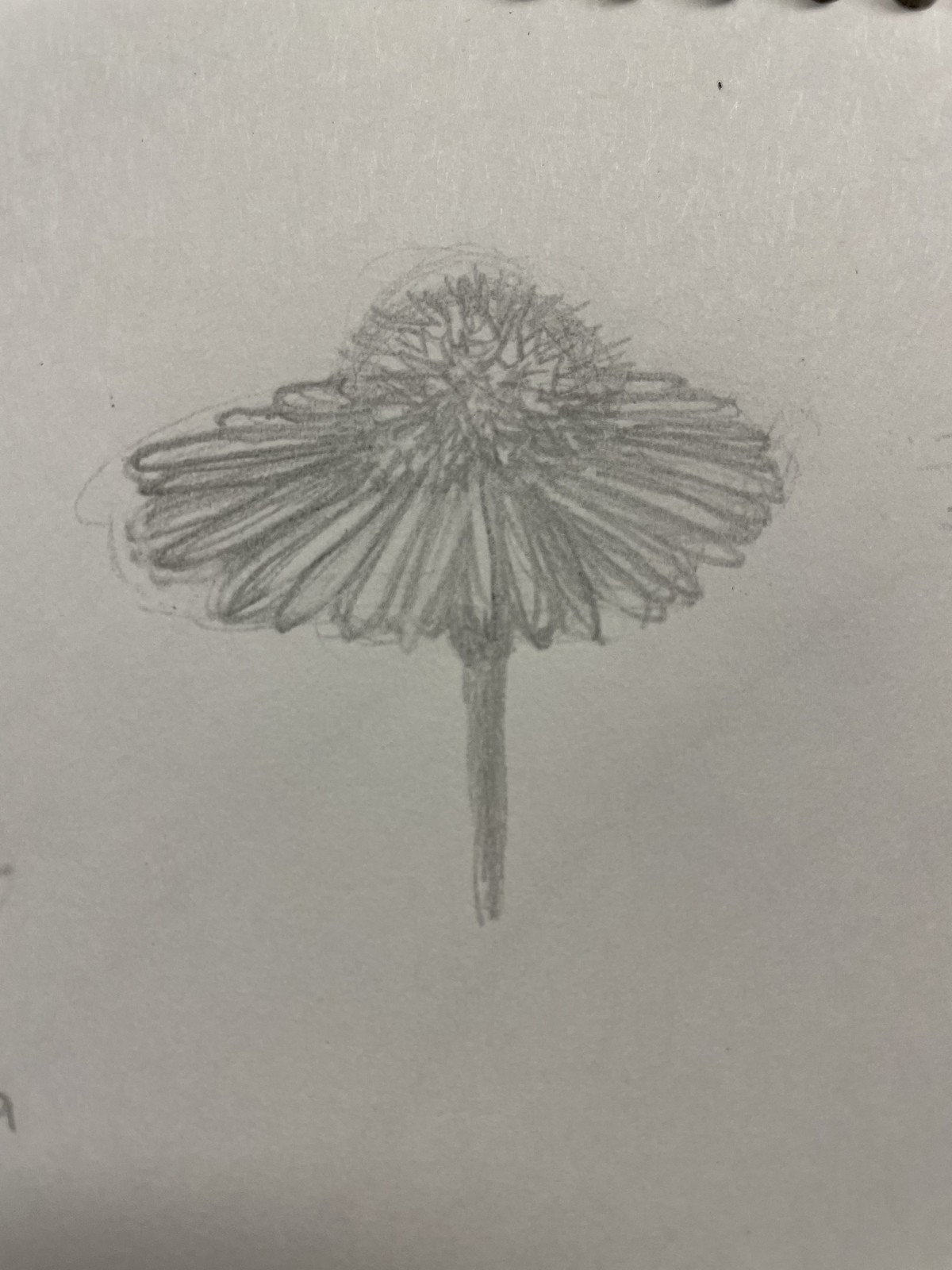This pencil drawing features a delicate flower with white petals radiating gracefully from its center. The upper part of the illustration subtly includes grassy elements, blending seamlessly with the petals to create a textured and natural appearance. The background is kept minimalistic, with a pristine white backdrop enhancing the flower's elegance and simplicity. The bottom of the image also features white, maintaining a cohesive, clean aesthetic throughout the entire piece.